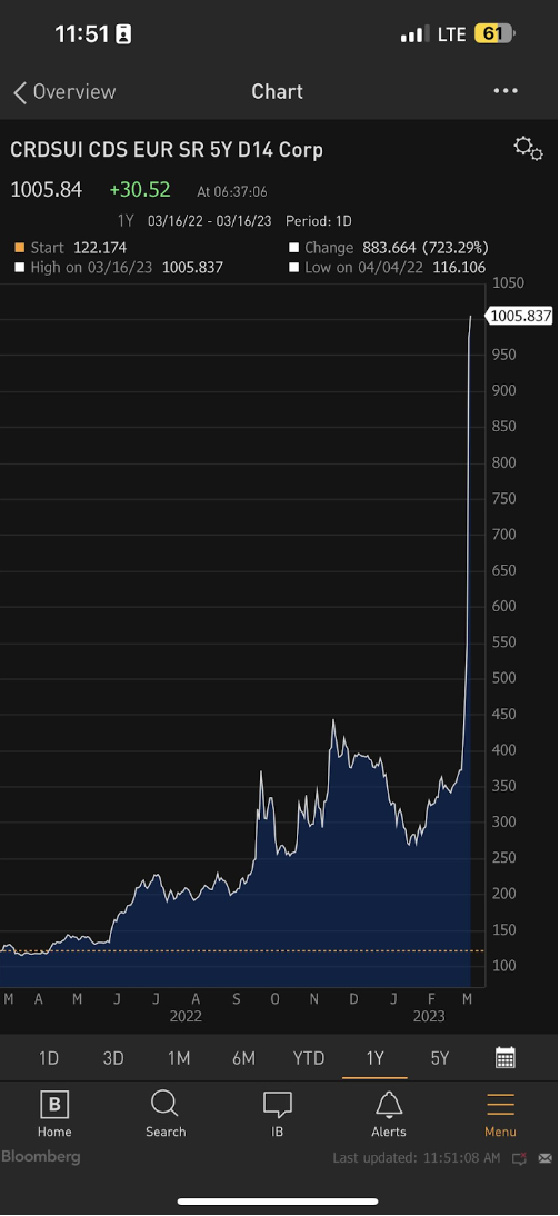The image depicts a screenshot of a stock market app displayed on a smartphone. In the top-right corner, the battery percentage is shown at 61%, with the battery icon in yellow, indicating that the device is in low power mode. The signal strength icon shows 3 out of 4 bars, and the connection type is LTE. On the left side of the top bar, the time is displayed as 11:51. 

The app interface features a dark grey banner at the top, labeled "Chart" in white text. To the right of this title are three dots, likely representing a menu for additional options, and to the left is an "Overview" button. Beneath this banner, the app focuses on a specific company, displaying stock prices against a timeline segmented into months, with values reaching up to 1005. 

At the bottom of the screen, there are navigation options including "Home," "Search," "IV Alerts," and a "Menu" button. Additional time frame options are available for viewing the stock data across different periods, such as yearly, five-year, yearly, monthly, and daily intervals.